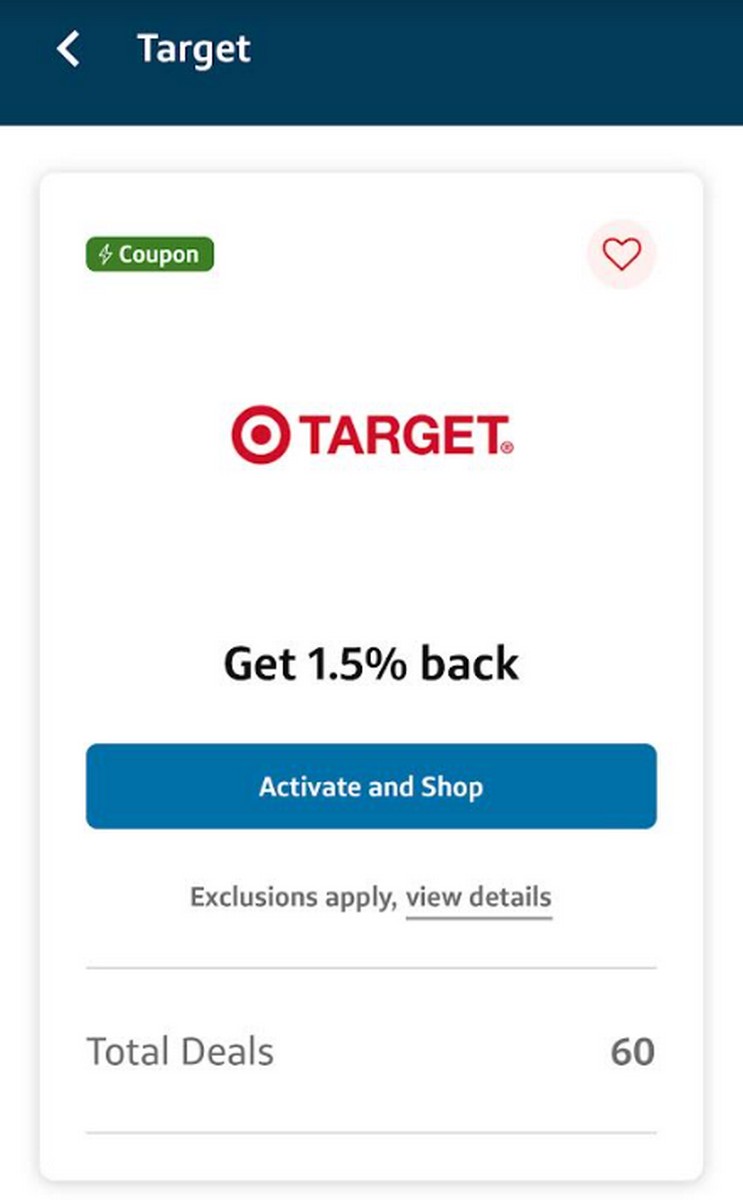This is a detailed caption for an image of a smartphone screenshot displaying a page on a shopping app:

---

The screenshot depicts a page from a shopping app, showcasing a section dedicated to Target. The background is navy blue, with the word "Target" prominently displayed in white text preceded by a less-than symbol (<). Below this, there's a long, white rectangle featuring a green triangle or rectangle in the upper left corner, adorned with a lightning bolt symbol and the word "Coupon" in white.

In the upper right corner of this white rectangle, there's a pale pink circle with a red heart inside it. Centrally positioned within the white rectangle is the Target logo, followed by the word "TARGET" in bold, capital letters. Directly below, in bold black text, it indicates "Get 1.5% back."

A blue banner beneath this text features a bold call-to-action button labeled "Activate and Shop." Following this, in smaller text, there is a note that says "Exclusions apply, view details," with "view details" underlined and rendered in gray.

A thin gray line divides this section from the next, where the words "Total deals" are listed alongside the number 60. Beyond a pale gray line at the bottom of the screenshot, the page concludes.

---